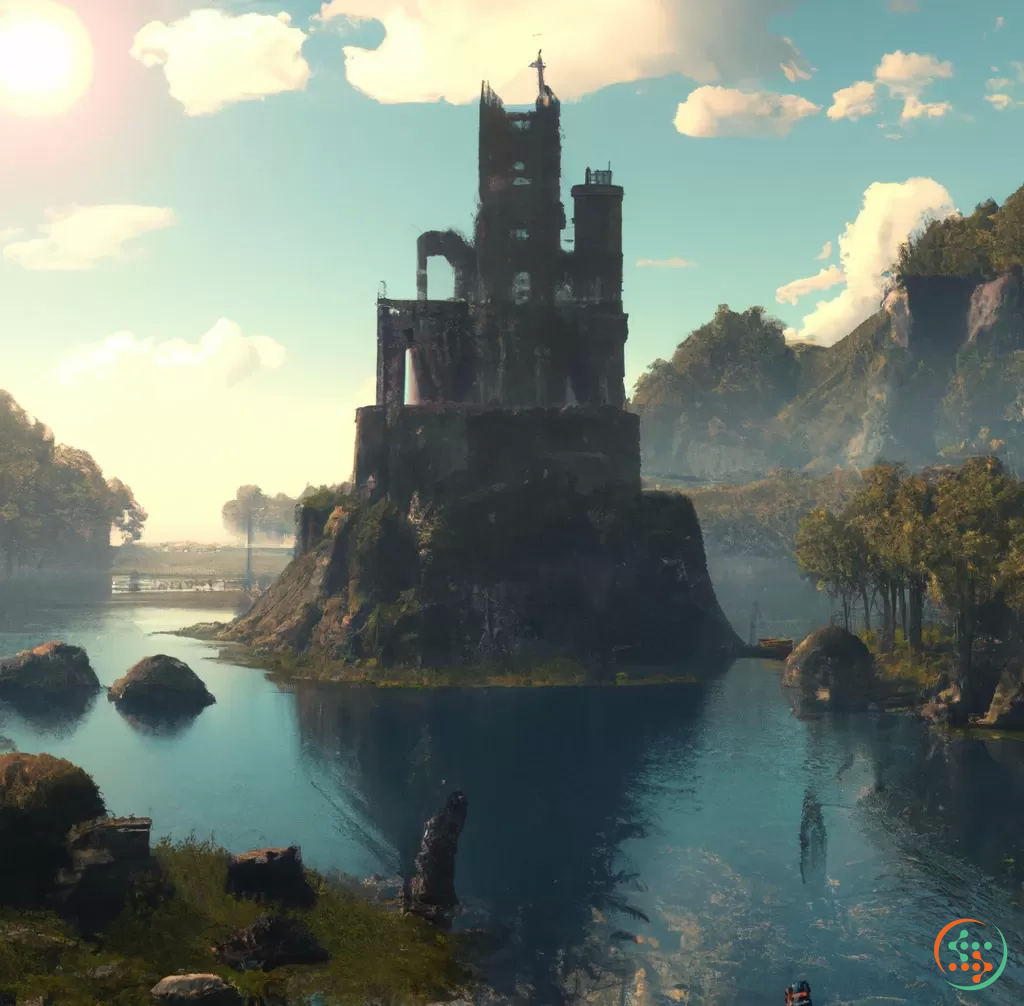This detailed image, reminiscent of a painting or computer-generated artwork, showcases a fantasy scene centered around a large, round island rising steeply from a bluish-green body of water that resembles a river. The island, surrounded by smaller rocks and landmasses with green trees and grass, is crowned by a majestic but decaying castle. The castle, which stands about three stories high, is primarily brown and gray, with hexagonal structures and tower elements. A prominent, tall rectangular section with a couple of windows sits at its center, while a smaller tower juts up from the right side. Water with bright blue ripples laps against the base of the island's steep rock walls. On the left bank, some grass can be seen, along with a person wading in the shallows. The background reveals distant rock hills, their slopes adorned with patches of greenery. Above, a light blue sky hosts thick white clouds tinted with gray, and a large bright sun in the upper left corner, encircled by a pale yellow halo, casts a serene, warm glow over the scene.